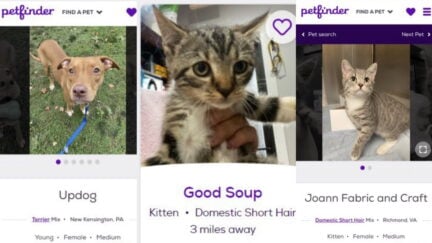This image collage features three distinct pet search results from Petfinder, showcasing adorable animals looking for loving homes:

1. The first image depicts a charming brown dog, tethered with a blue leash, standing alertly on a grassy lawn. His expressive eyes gaze up at the camera, radiating a sense of curiosity and sweetness.

2. The second image features a tiny domestic shorthair kitten, described as "Good Soup," located just three miles away. The kitten, approximately eight weeks old, has a soft gray and white coat. It appears to be at a veterinarian's office, as evidenced by the stethoscope visible in the background. The kitten rests gently in someone's hands, adding a touch of tenderness to the scene.

3. The final image is of another domestic shorthair kitten, lighter gray and white in color, and slightly different in shading compared to the previous kitten. This feline is being searched under "Joanna Fabric and Craft" and also appears to be at the same veterinary setting, given the consistent background elements.

Overall, these images, unified by Petfinder’s distinctive purple and white interface, capture the essence of these adorable pets—a loving brown dog and two precious kittens, each exuding their unique charm and eagerness to find a forever home.